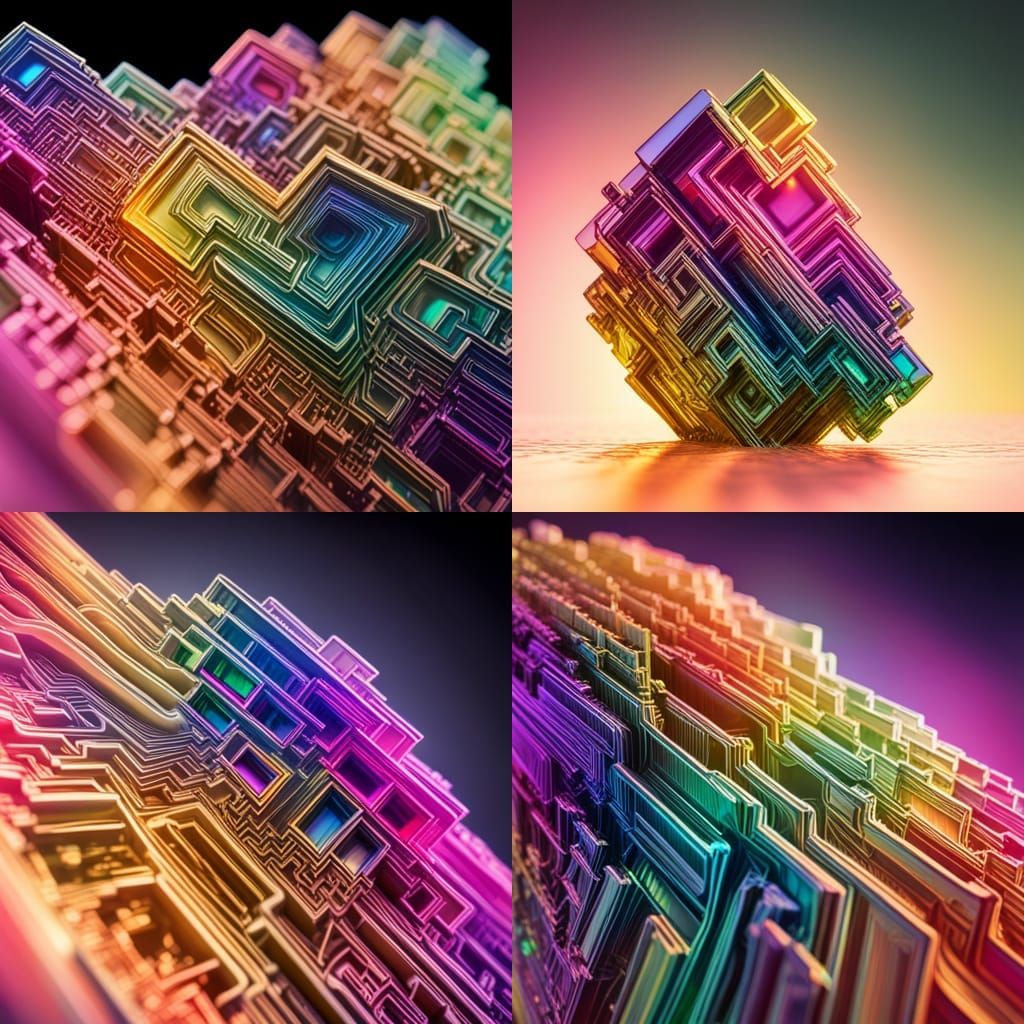This artwork is an AI-generated piece composed of four distinct, yet cohesive images, arranged in a grid with two images on top and two on the bottom. Each segment features a complex and layered design with various square edges and lines, resembling a labyrinthine structure. The intricate patterns form a neon rainbow aesthetic with vibrant fluorescent hues, including pinks, greens, blues, purples, yellows, and golds. 

In each image, the background color gradients range from black to vibrant colors like purple, yellow, green, and pink, emphasizing the futuristic and otherworldly feel of the piece. The top-left image displays a black backdrop with a maze-like square and line design in multiple colors, creating a striking contrast. The top-right image has a purple to yellow-green gradient background with a glowing yellowish floor, featuring a central diamond-shaped artwork that mirrors the square-line pattern.

The bottom-left image presents a dark purple background fading to black, with a flat depiction of the intricate maze design in neon colors. The bottom-right image, set against a pink to black gradient backdrop, portrays a structure resembling a stack of folders, coated with the same colored square and line pattern. Together, these images blend into a harmonious yet vivid composition, showcasing the capabilities of AI in generating intricate, colorful, and visually captivating designs.